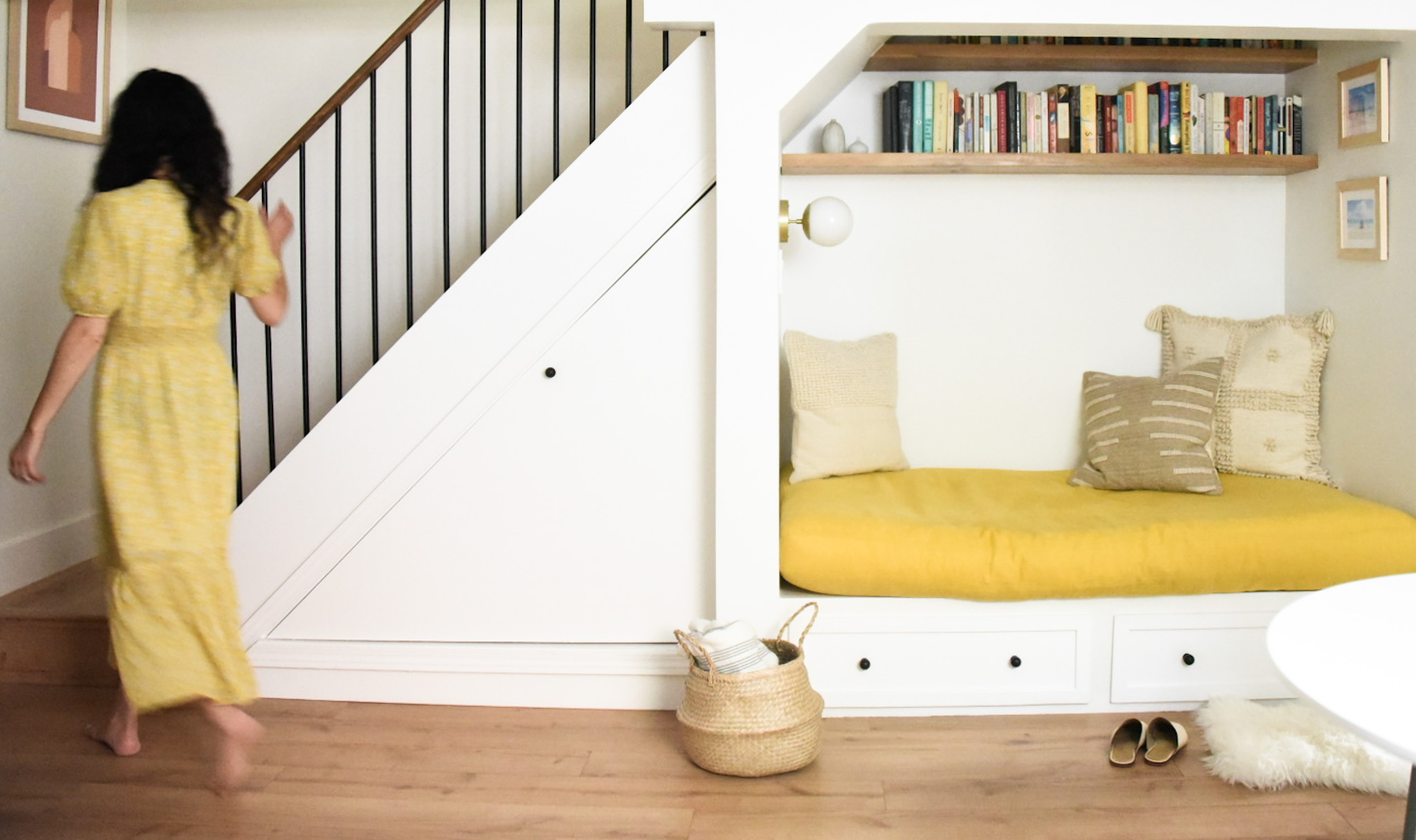In this cozy indoor scene, a woman with medium-length dark brown wavy hair is captured walking barefoot towards a white staircase on the left side of the image. She is dressed in a long, flowing yellow sundress. The staircase, which ascends to the upper level of the home, has an inviting nook beneath it. This reading nook features a large yellow cushion with three throw pillows, creating a perfect relaxation spot. Above the cushion, a pair of shelves is adorned with a variety of books and softly lit by an installed light. A couple of pictures decorate the wall, enhancing the charm of the space. A fuzzy white rug lies on the floor beside the nook, along with a pair of house shoes and a basket holding white towels. This serene setting implies the woman may have been sitting and reading there before deciding to head upstairs.